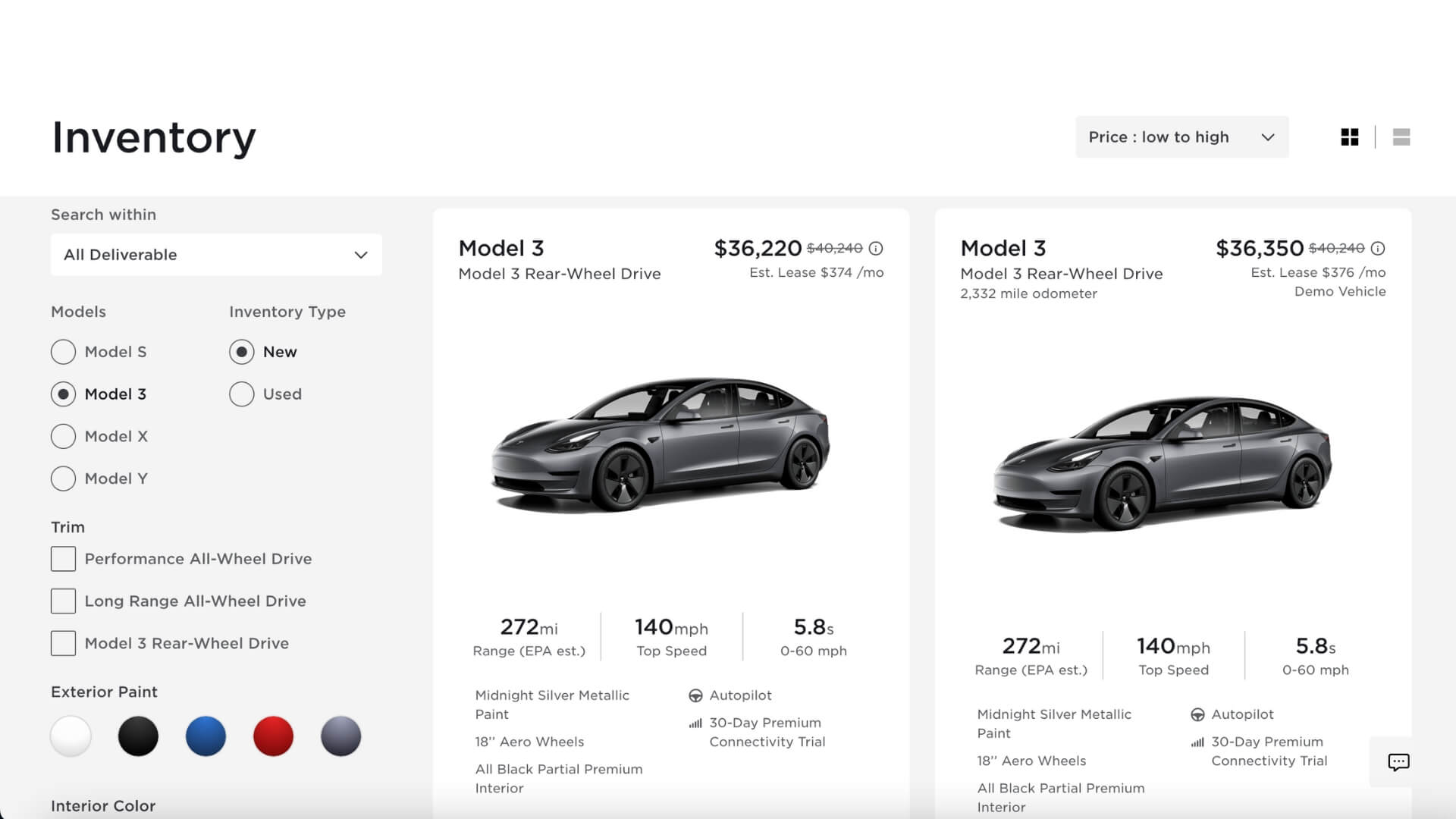A screenshot displays a detailed inventory interface, likely from an automotive website, showing a Tesla vehicle selection process. In the upper left corner, "Inventory" is prominently visible, with a "Price: Low to High" dropdown menu to its right, followed by several navigation or sorting options. 

On the left side of the screen, a search filter section is present. It includes a "Search Within" dropdown currently set to "All Deliverables." Below, a list of Tesla vehicle models is shown, with "Model S," "Model 3" (selected), "Model X," and "Model Y" as radio button options. Adjacent to this, the "Inventory Type" section features "New" and "Used" options, with "New" selected. Another filter category, "Trim," lists options such as "Performance All-Wheel Drive," "Long Range All-Wheel Drive," and "Model 3 Rear-Wheel Drive," all depicted through checkboxes. 

Further down, an "Exterior Paint" section offers various selectable colors, followed by an "Interior Color" section, which is partially cut off in the screenshot.

In the central-right section of the screen, two comparable car listings are displayed side-by-side. Both are "Model 3" with "Rear-Wheel Drive" trim. The left car is priced at $36,220, crossed out from $40,240, and includes details like mileage range and top speed. The right car appears nearly identical but does not list a 2.332-mile odometer reading.